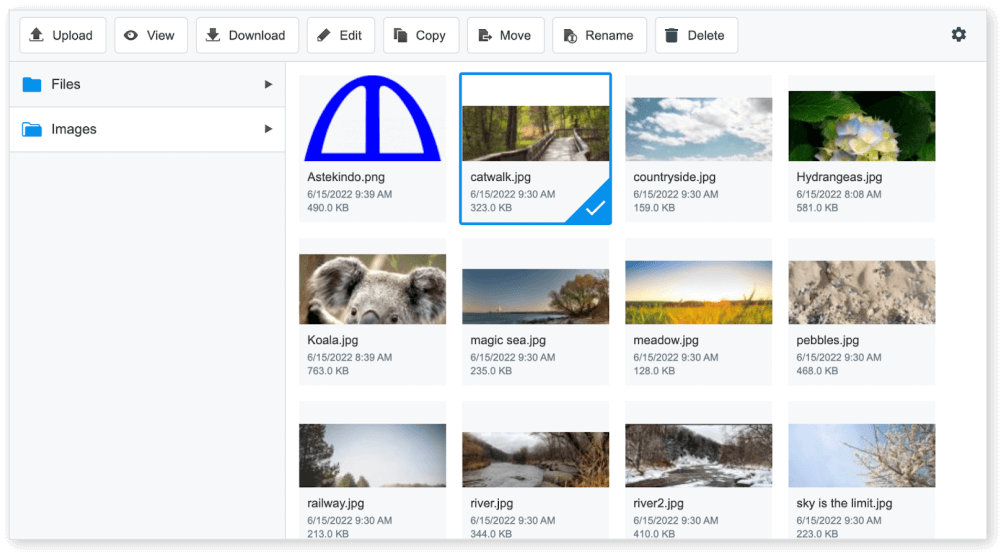A detailed screenshot of a web browser with nine tabs open is depicted, representing various file management actions: Upload, View, Download, Edit, Copy, Move, Rename, and Delete. The left pane features two sections labeled 'Files' and 'Images', each marked with blue folder icons.

On the right pane, set against a white background, twelve individual photographs are displayed. Each photograph is distinct, accompanied by its filename, format (NPG or JPG), date, time of capture, and file size.

The first image portrays a Blue Arch, titled "Aztecindo.png", captured on 5-15-2022 at 9:39 AM, with a size of 490 KB. The second image features a bridge in a forest, named "catwalk.jpg", taken on 6-5-2022 at 9:30 AM, with a size of 323 KB. This image is highlighted with a blue border and has a checkmark at its bottom-right corner.

The third image shows clouds, labeled "countryside.jpg", dated 6-5-2022 at 9:30 AM, with a file size of 159 KB. The fourth image in the first row is of blue and white hydrangeas with green foliage, titled "hydrangeas.jpg", captured on 6-5-2022 at 8:08 AM, and sized at 581 KB.

Additional photographs displayed primarily showcase nature and landscapes, with one featuring an animal. These images add to the visual richness of the right pane, collectively representing a diverse array of subjects.